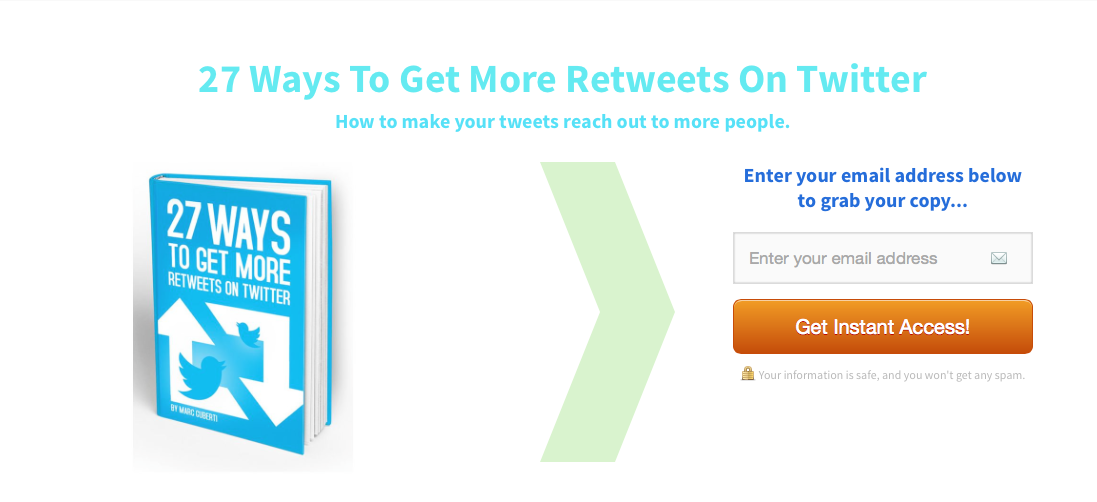The image depicts a webpage dedicated to promoting an upcoming book titled "27 Ways to Get More Retweets on Twitter: How to Make Your Tweets Reach Out to More People." The book, prominently displayed on the left side of the page, features a blue cover with white lettering. The title "27 Ways to Get More Retweets on Twitter" is clearly visible, accompanied by circling arrows and blue Twitter birds that adorn the cover, emphasizing the social media theme. Although the author's name is written at the bottom of the cover, it is not distinguishable in the image.

On the right side of the webpage, there is a call-to-action prompting visitors to enter their email address to receive a copy of the book. Below this prompt, a text box is provided for email entry, marked with a small email icon. Beneath the text box, a prominent orange button with the text "Get Instant Access!" catches the eye, encouraging immediate interaction. At the bottom of the page, a small lock symbol paired with fine print assures users that their information is safe and guarantees that they will not receive any spam.